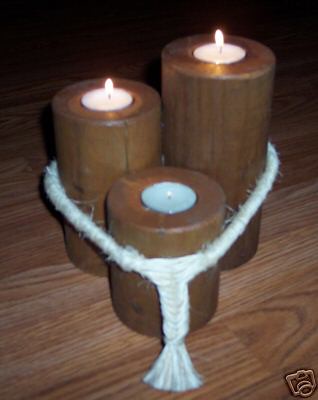The photo, though not of the best quality, depicts three brown wooden pillar-style candle holders on a faux wood surface, possibly a countertop or floor. Each pillar holds a white tea light candle at varying heights. The tallest candle holder is positioned on the upper right, the mid-sized one is to the left, and the shortest is in front. All three tea light candles are lit, with the tallest and mid-sized showing a robust flame, while the shortest has a flame that appears to be barely flickering and about to go out. The three candle holders are bound together with a piece of white rope tied in front, highlighting their unity. Additionally, an indistinct insignia, possibly a square with two circles, is visible in the bottom right-hand corner of the image. The background reveals a darkened, rich brown wood, adding depth to the composition.